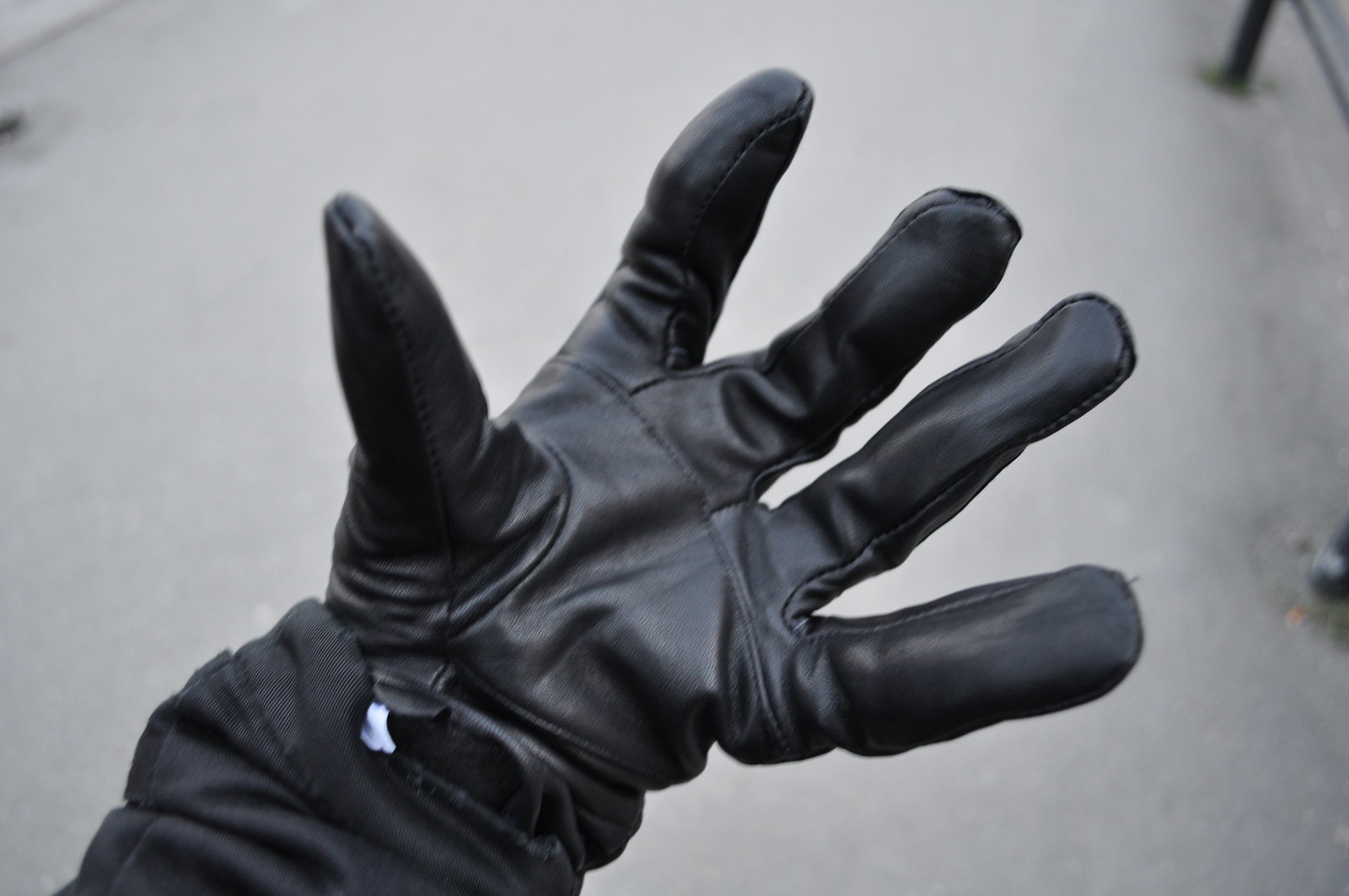In this black and white photograph, the main focus is a gloved left hand extending upward from the bottom left side of the image. The glove, which appears to be either vinyl or leather, is black and somewhat bulky, with the palm outstretched as if ready to catch something. Just peeking below the glove, a small white tag is visible, and the person is wearing a black coat or jacket, possibly a ski jacket. The background is a uniform white, with a blurred gray floor or wall extending across the frame. In the top right corner, a black pole and a silver object are visible, though they are not the main subject, adding a subtle hint of context to the overall composition.